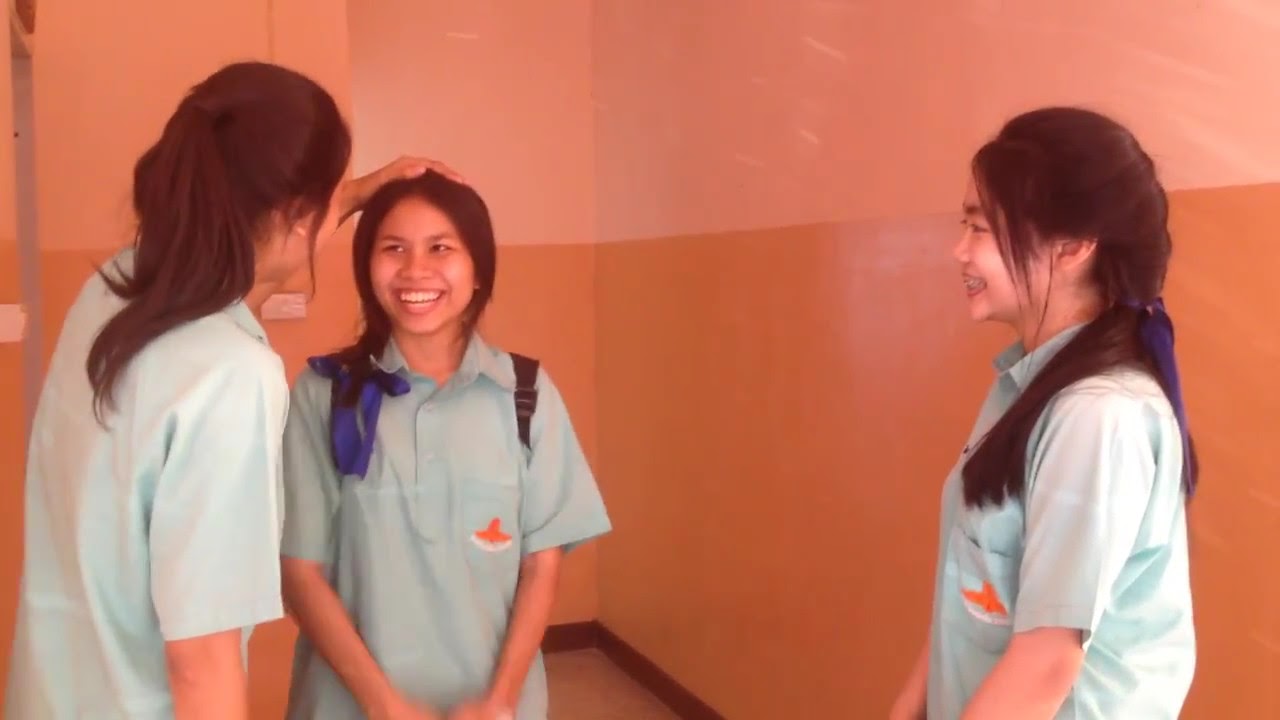In this horizontally aligned rectangular picture, three young women stand together in a corner of the room, set against a two-toned wall — the bottom half is orange and the top half is pink. The background is somewhat blurry, with a visible doorway on the left. All three women have long, straight, dark brown hair pulled back, and they are wearing the same light blue collared button-down shirt with an orange logo on the left chest, suggesting a uniform, possibly for a professional or educational setting.

On the left side, one of the women, seen from the right and back, has her hair pulled into a ponytail and is looking at the woman standing next to her. This second woman, who is also on the left, has her hair similarly styled and is smiling broadly, with teeth showing, and a shoulder strap from either a backpack or a purse draped over her left shoulder.

Further to the right stands the third woman, a bit apart from the other two. She is smiling widely, showing her braces. Her hair is pulled back, and she too is wearing the uniform shirt. Her left hand is raised to her head, adding a casual, playful element to the scene. Their expressions and body language suggest a moment of shared joy and camaraderie, captured within the vibrant orange and pink hues of the room.

Overall, the image conveys a lively and cheerful atmosphere, characterized by the vibrant background and the trio's coordinating outfits and cheerful expressions.